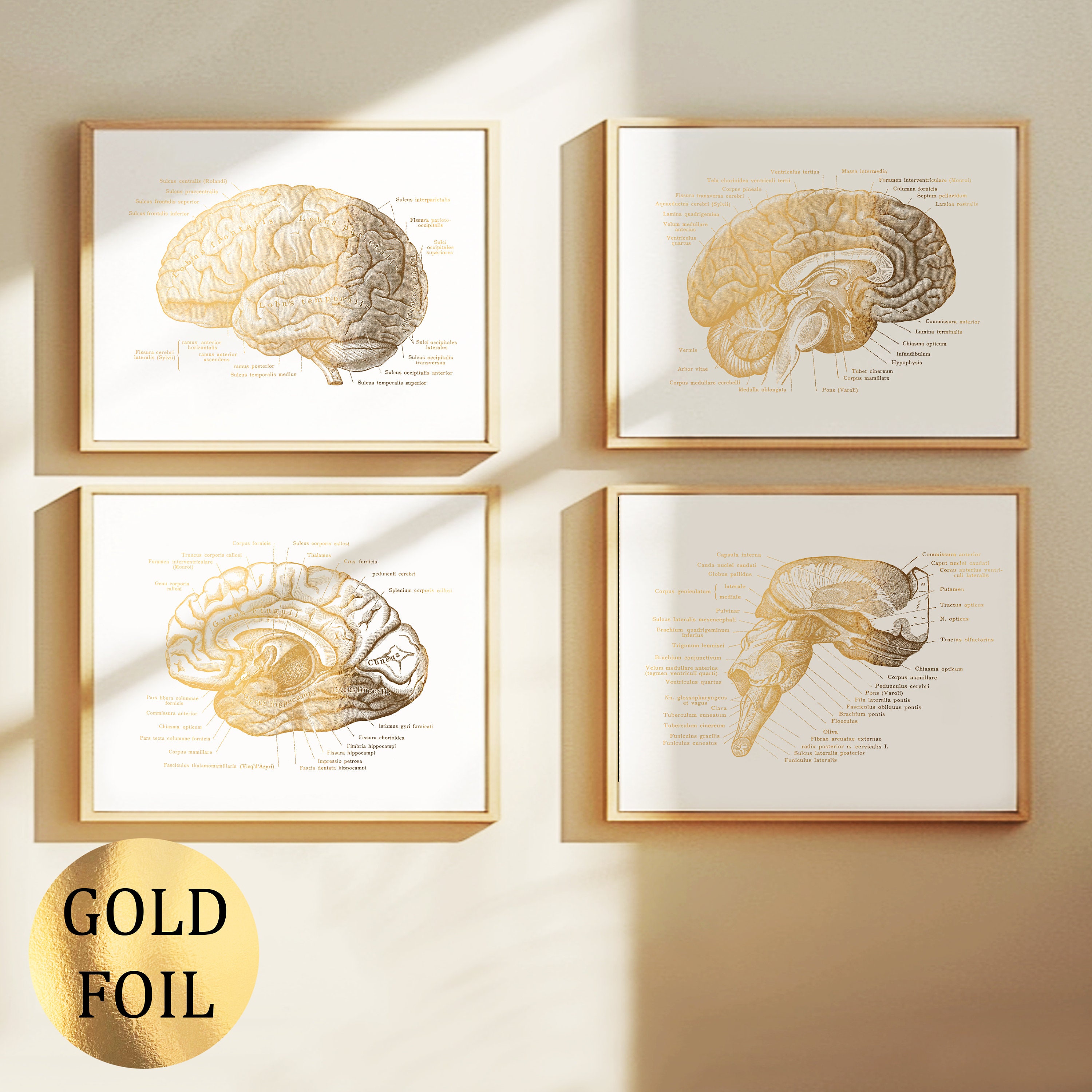The image showcases four wooden-framed, hand-drawn illustrations of the human brain, each depicting different cross-sections labeled in brown ink against a white background. These framed medical diagrams, all identical in size and style, are arranged on a beige wall. Sunlight streaming in from the left casts a warm glow on the leftmost illustrations while the right two are partly shrouded in shadow, revealing the possible outline of a window. A notable feature is a gold foil circle with black text that reads "gold foil" positioned at the bottom left corner, which seems to be an additional label distinct from the brain illustrations. Overall, the scene blends elements of scientific precision with aesthetic wall art, enhanced by natural light.